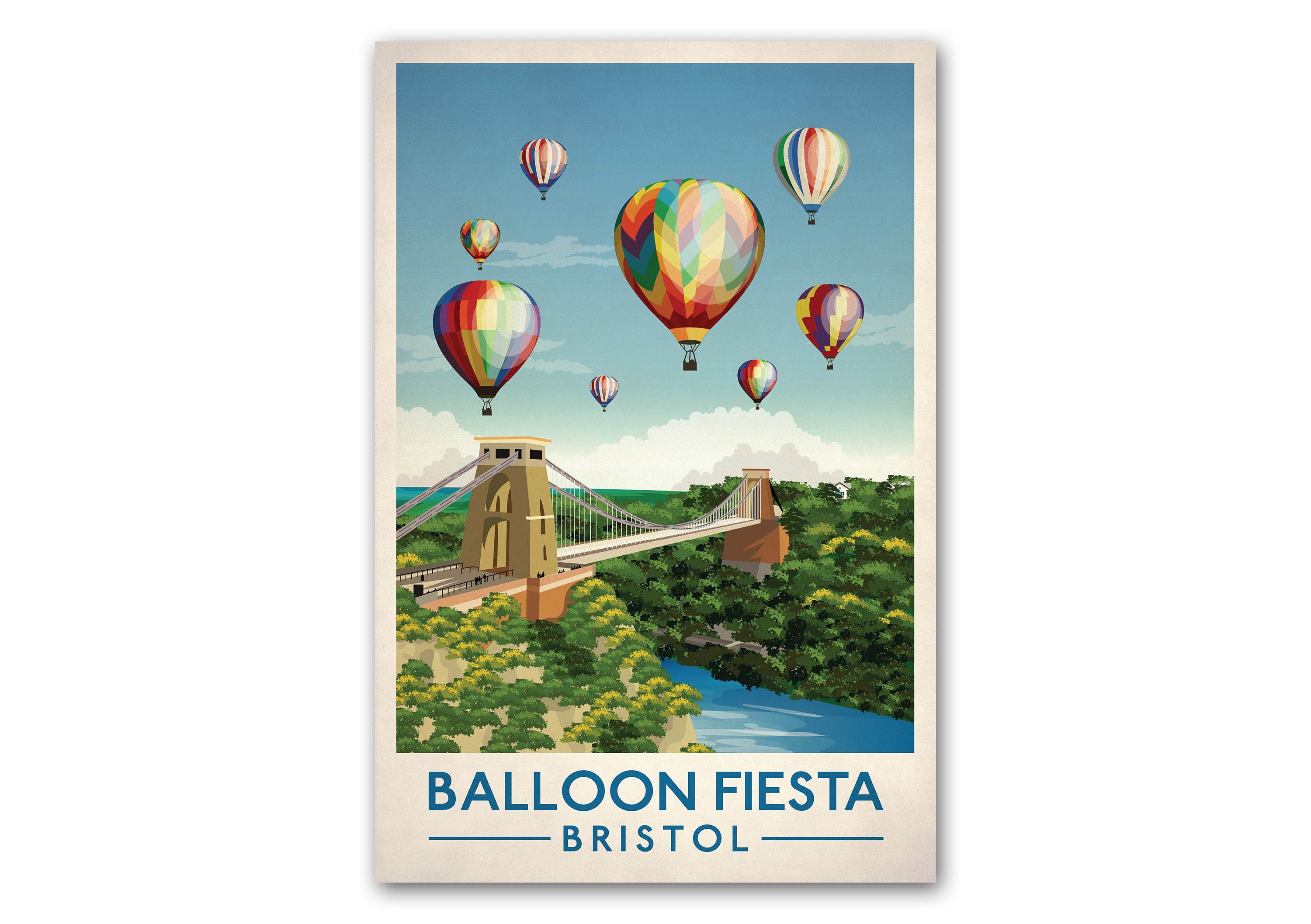This image is a detailed watercolor-style illustration from a magazine, serving as an advertising poster for the Balloon Fiesta in Bristol. The artwork features a suspension bridge that resembles a shorter version of the Golden Gate or Brooklyn Bridge, painted in shades of reddish-brown, orange, and tan sandstone. The bridge spans a river or large valley, with its clear blue water reflecting the bright sky above, dotted with scattered white clouds.

In the centerpiece of the image, eight hot air balloons of various sizes drift above the bridge. These balloons boast a rainbow of colors—reds, blues, greens, yellows, and purples—decorated with patterns such as stripes and chevrons. The balloons are positioned at different distances, giving a sense of depth and scale to the scene.

The landscape around the bridge is lush with vegetation, including green bushes and yellow flowers covering the hillsides. The entire illustration is framed by a white border, with the caption "Balloon Fiesta, Bristol" in blue text at the bottom, completing this vibrant and whimsical depiction of a festive event.